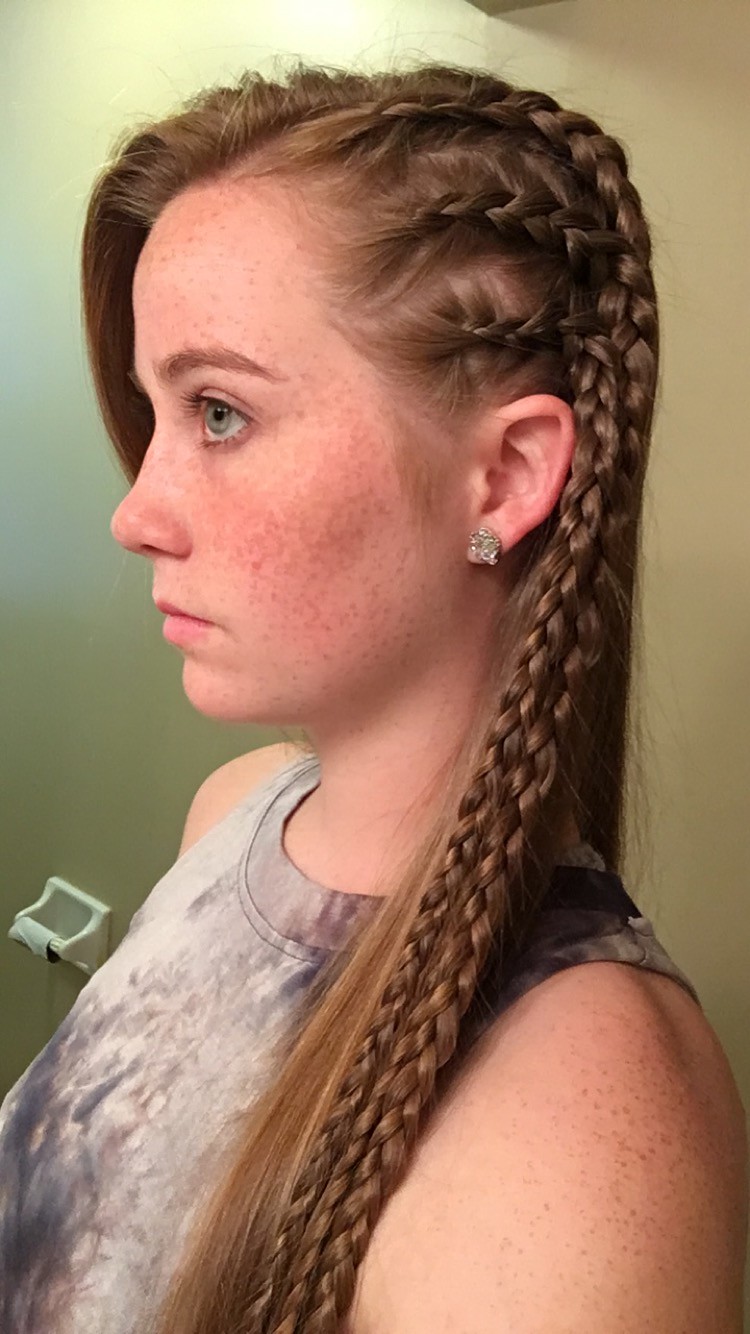This is a detailed photograph of a young woman, approximately in her late teens to mid-20s, with a blend of reddish-brown or brown hair styled in intricate French or Dutch braids. Her hair, parted and tightly braided close to her scalp, trails down over her shoulder in multiple strands, leaving some natural hair untouched on one side. She has light green or grayish-green eyes, delicate freckles matching her hair color, and wears a prominent, sparkly, silver diamond-like earring. The young woman is dressed in a sleeveless top with a dirty purple or grayish tie-dye pattern. The image captures her from the side profile, gazing off to the left, with a white wall behind her suggesting an indoor, possibly bathroom setting as indicated by the visible toilet paper dispenser. Her expression appears frozen, possibly indicating discomfort or tension.